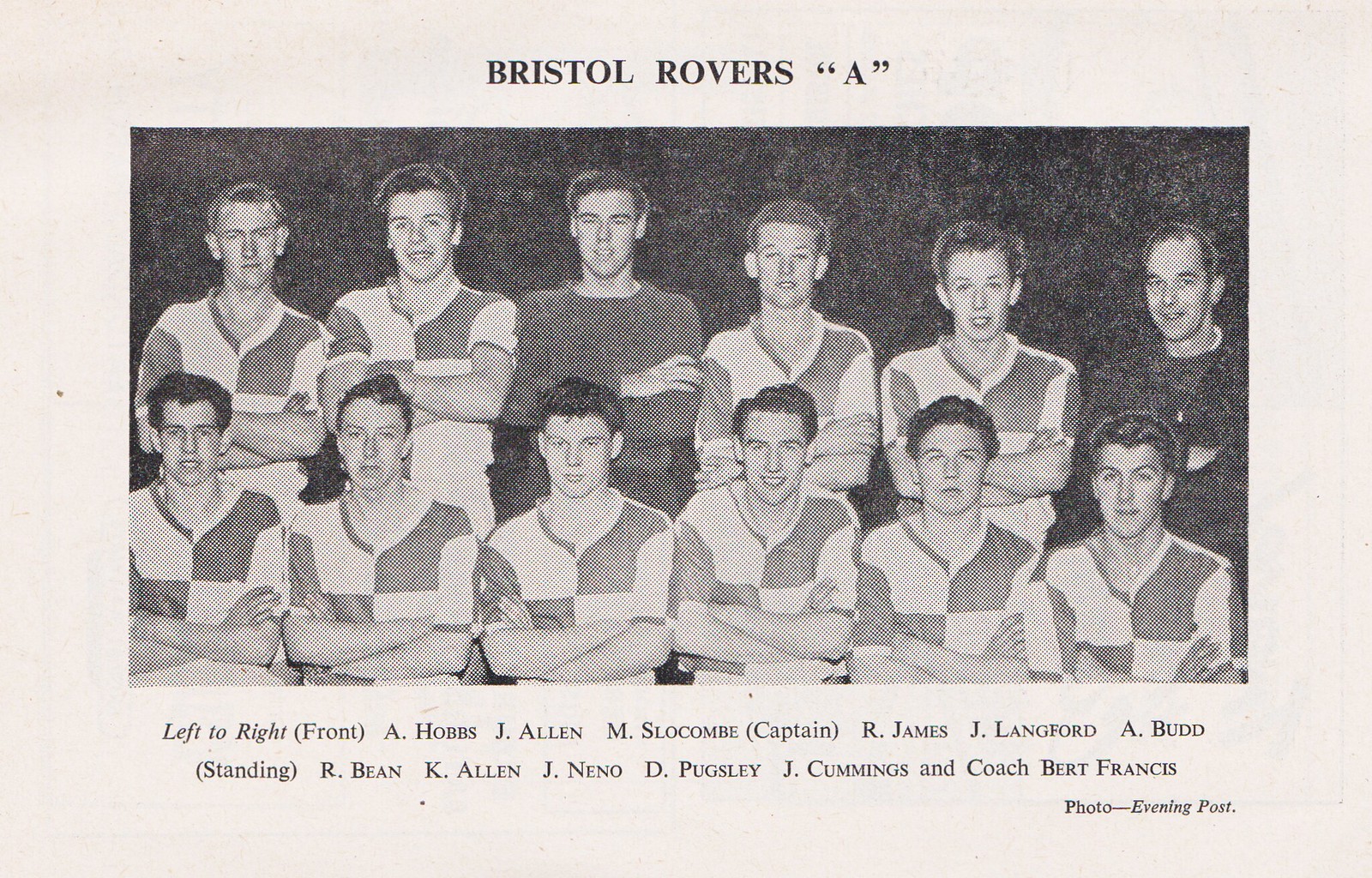This black and white, grainy, and slightly faded photo captures a vintage soccer team from possibly the 50s or 60s. At the top, a title reads "Bristol Rovers 'A'." The team is arranged in two rows: six men standing in the back and six seated in the front. Most players are donning large checkered jerseys, though two wear solid-colored tops. All the men have their arms crossed, with expressions ranging from slight smiles to more solemn looks. Below the image, the caption is detailed: "Left to right, front: A. Hobbs, J. Allen, M. Slocum (Captain), R. James, J. Langford, A. Budd. Standing: R. Bean, K. Allen, J. Nino, D. Pugsley, J. Cummings, and Coach Bert Francis." The annotation further notes "Photo: Evening Post."